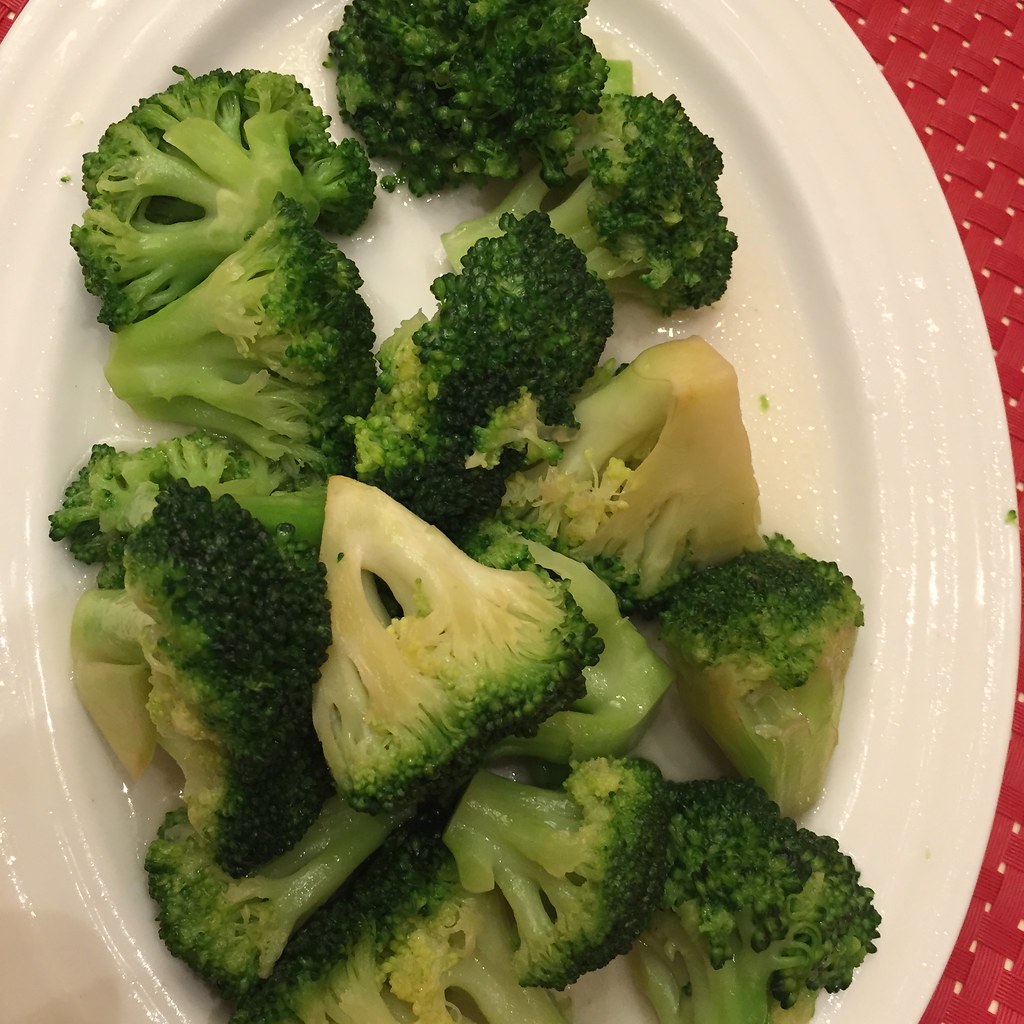This indoor color photograph features a white, oval ceramic plate filled with approximately 15 to 16 broccoli florets. The plate is placed on a red and white checkered placemat, visible in the lower right and upper right corners of the image. The camera is positioned directly above the plate, capturing the textured surface of the placemat, which has a red woven material amidst a white background with tiny specks.

The broccoli florets, displaying a deep, dark green color at the top transitioning to a lighter green on the stems, appear to be steamed or cooked, with some droplets of water, sauce, or butter visible on them. The florets fill almost the entire plate, some arranged along the edges, with a few pieces facing downward into the plate. One notable piece in the center is lighter in color. The meticulous arrangement and untouched appearance of the broccoli suggest that it has just been served. The entire image is free of any text or wording, focusing solely on the visual presentation of the dish.